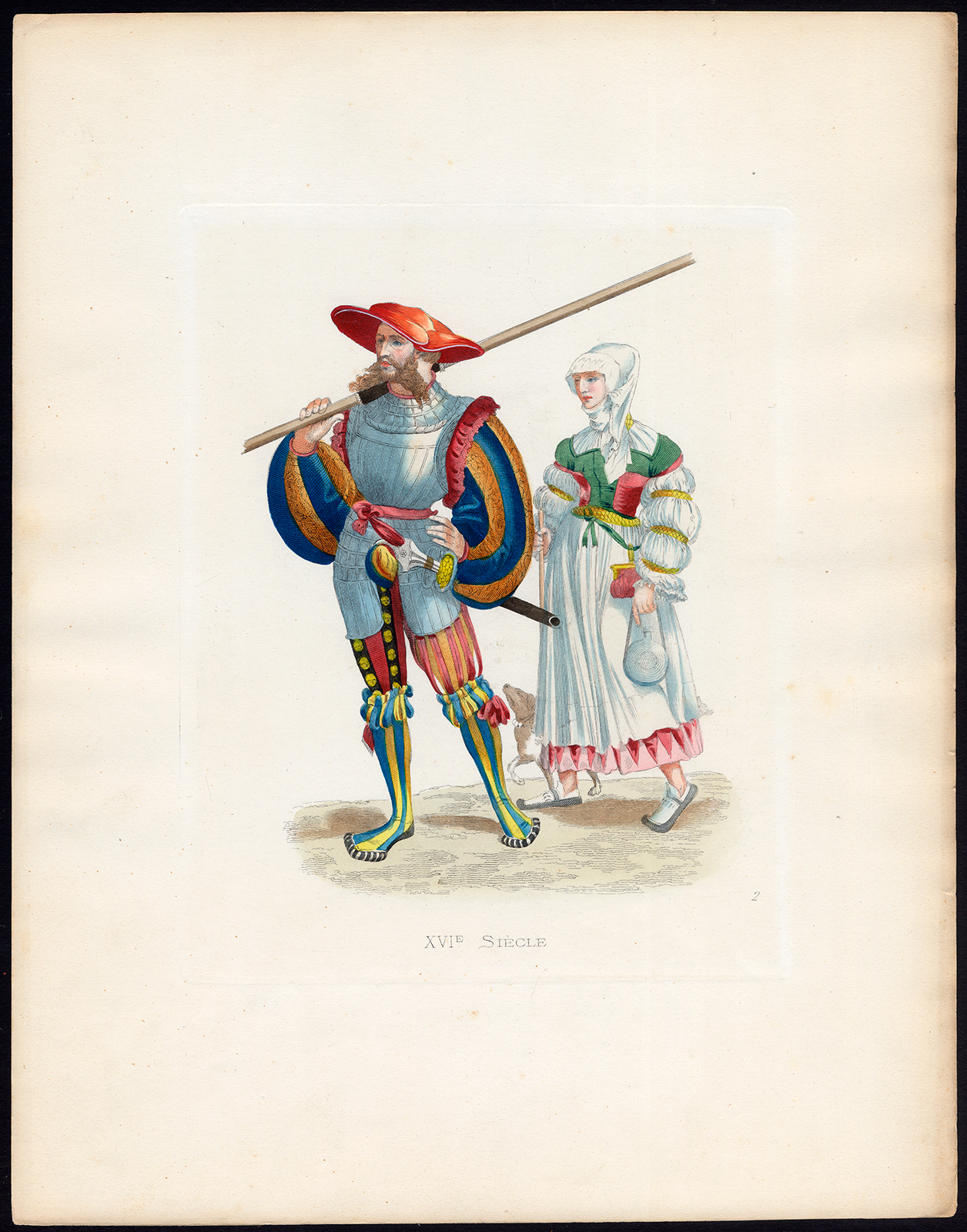This detailed Renaissance-era illustration, enclosed in a thin black frame on a yellowed paper backing, portrays a knight standing left-center with a lady behind him. The knight, perhaps also evoking a jester’s attire, wears a red floppy hat atop his brown beard. His torso is armored in silver from his neck to his upper thighs, complemented by billowy orange and blue striped sleeves with red accents. His lower thighs are clad in vivid red and yellow striped fabric, while his knee-high socks feature a turquoise, blue, and yellow stripe pattern. He holds a pole over his shoulders. The lady beside him dons a white headpiece and a white gown with a green bodice and red ruffle trim. Her outfit includes billowy sleeves and a skirt revealing a pink slip above her ankles, paired with flat white shoes with gray soles. They stand on a checkered white and dark pavement, with unreadable text beneath. The lady holds a circular canteen, echoing the medieval aesthetic.